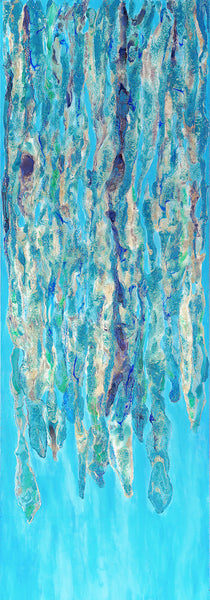The image depicts a very tall and narrow abstract painting with a predominantly bright turquoise blue background, which becomes more visible towards the bottom of the picture. The composition is characterized by various streaks and blobs that cascade from the top to nearly the bottom of the image, resembling icicles or water droplets. These formations are expressed through distinct, bold brushstrokes in shades of blue — including light blue, dark blue, and navy — as well as some hints of beige and gray. The streaks and blobs in the center are primarily blue, with the largest being a dark blue that showcases prominent brushstrokes. The scraggly, overlapping strokes create a sense of drips or vines hanging down. There is no text within the image, which embodies the qualities of modern abstract art, merging elements that evoke natural crystalline structures or cave stalactites. The intricate interplay of colors and lines on the turquoise blue backdrop defines its dynamic and somewhat chaotic aesthetic.